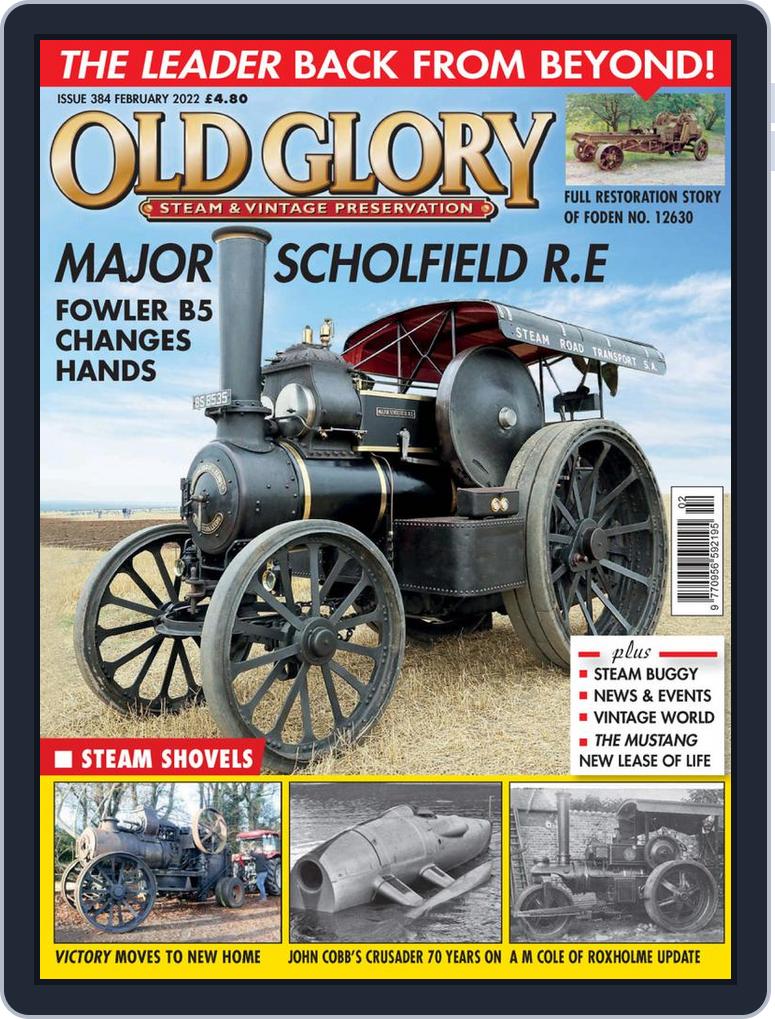This cover of the magazine "Old Glory Steam and Vintage Preservation," Issue No. 384, February 2022, priced at $4.00, captivates enthusiasts of vintage steam-powered machinery. Dominated by a striking image of an early 1900s steam-powered vehicle, the central feature showcases a meticulously restored machine with a round, black steam engine, a prominent smokestack, and rubber-coated wagon-style wheels—smaller in the front and larger in the back. The cover highlights the full restoration story of "Foden No. 12630," as indicated in the upper right corner, and announces the ownership change of "Major Schofield RE, Foul or B5."

The red banner at the top reads, "The Leader Back From Beyond," emphasizing the return of significant vintage steam technology. Below this, additional articles are prominently advertised: "Steam Shovels: Victory Moves to New Home" features a large, complex steam-powered machine; "John Combs Crusader: 70 Years On" shows a partially submerged, possibly flood-damaged vehicle; and "A.M. Cole of Rocks Home Update" depicts another similar steam-powered vehicle.

A white box with black lettering announces, "Steam Buggy, News and Events, Vintage World, The Mustang, New Lease on Life," further diversifying the magazine's rich content. The meticulous detail and vibrant history captured in this issue make it a treasure trove for steam machinery aficionados.